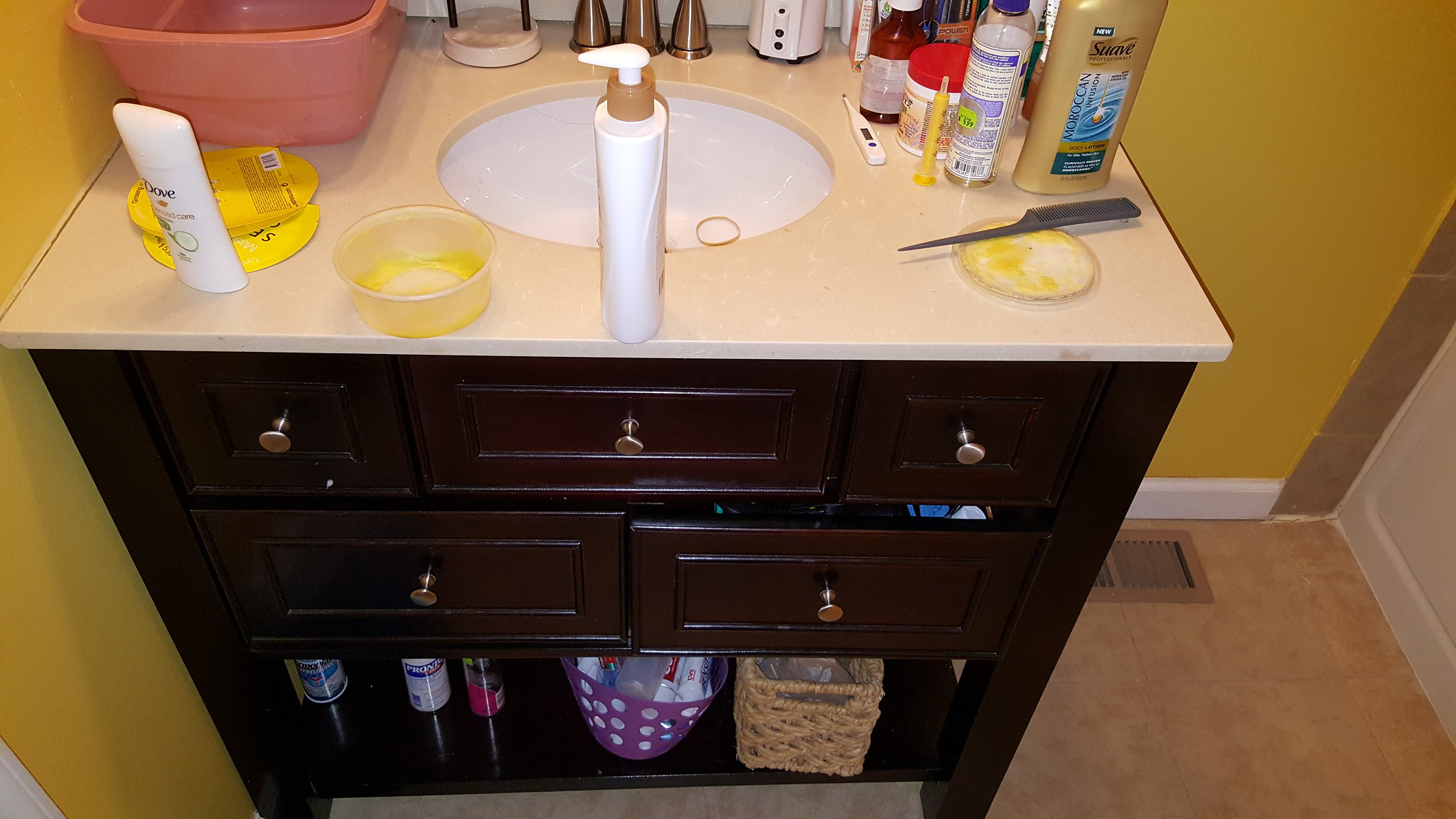The photograph captures a well-detailed view of a bathroom. The walls are painted a vibrant yellow, complemented by white trim along the base near the floor. The flooring consists of square brown tiles that add a rustic touch to the room. In the back right corner of the floor, there is a brown painted vent, presumably for a heating duct. To the right, the edge of a white wall or possibly a door is partially visible, slightly cut off by the frame.

Prominently in the foreground stands a dark brown cabinet. The bottom shelf of the cabinet holds a wicker basket, a purple plastic basket perforated with holes containing what appears to be toothpaste and other items, and a couple of cans whose labels are not visible. Above this open shelf are five drawers: three arranged in a rectangular formation and two in square shape, each adorned with silver pulls.

Atop the cabinet sits a sink with a white marble countertop featuring an off-white hue, contrasting with the pure white basin. The left side of the countertop houses a Dove deodorant stick. An empty canister with a yellow residue, likely hair gel, and its lid rests on the right side. Scattered across the countertop are also a gray comb, a bottle of Suave shampoo, and a thermometer, adding to the lived-in feel of the space.